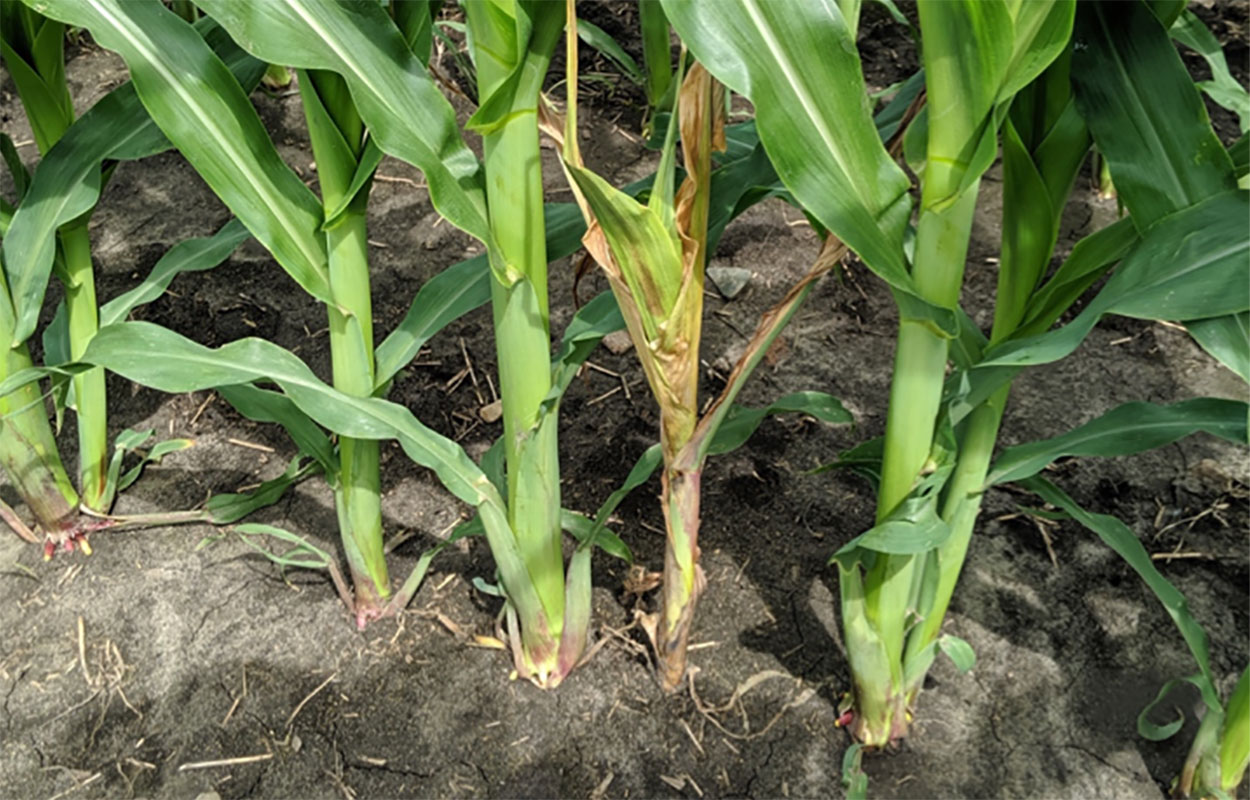The photograph, rectangular in shape with its length twice that of its width, captures a detailed view of a neat row of corn stalks against a backdrop of dark brown soil. The focal point is the six corn stalks arranged in a row, where five of them appear healthy with a vibrant green color, indicative of well-nourished plants. The sixth stalk, prominently positioned in the center, starkly contrasts with the others, as it is yellowed and brown, showing signs of stunted and irregular growth. The soil appears moist, suggesting recent irrigation, and is dotted with various strands of roots and scattered fallen vegetation. Shadows fall across the ground, emphasizing the depth and texture of the soil, which also contains some rocks. The absence of weeds indicates meticulous care taken in maintaining this small section of a larger crop.